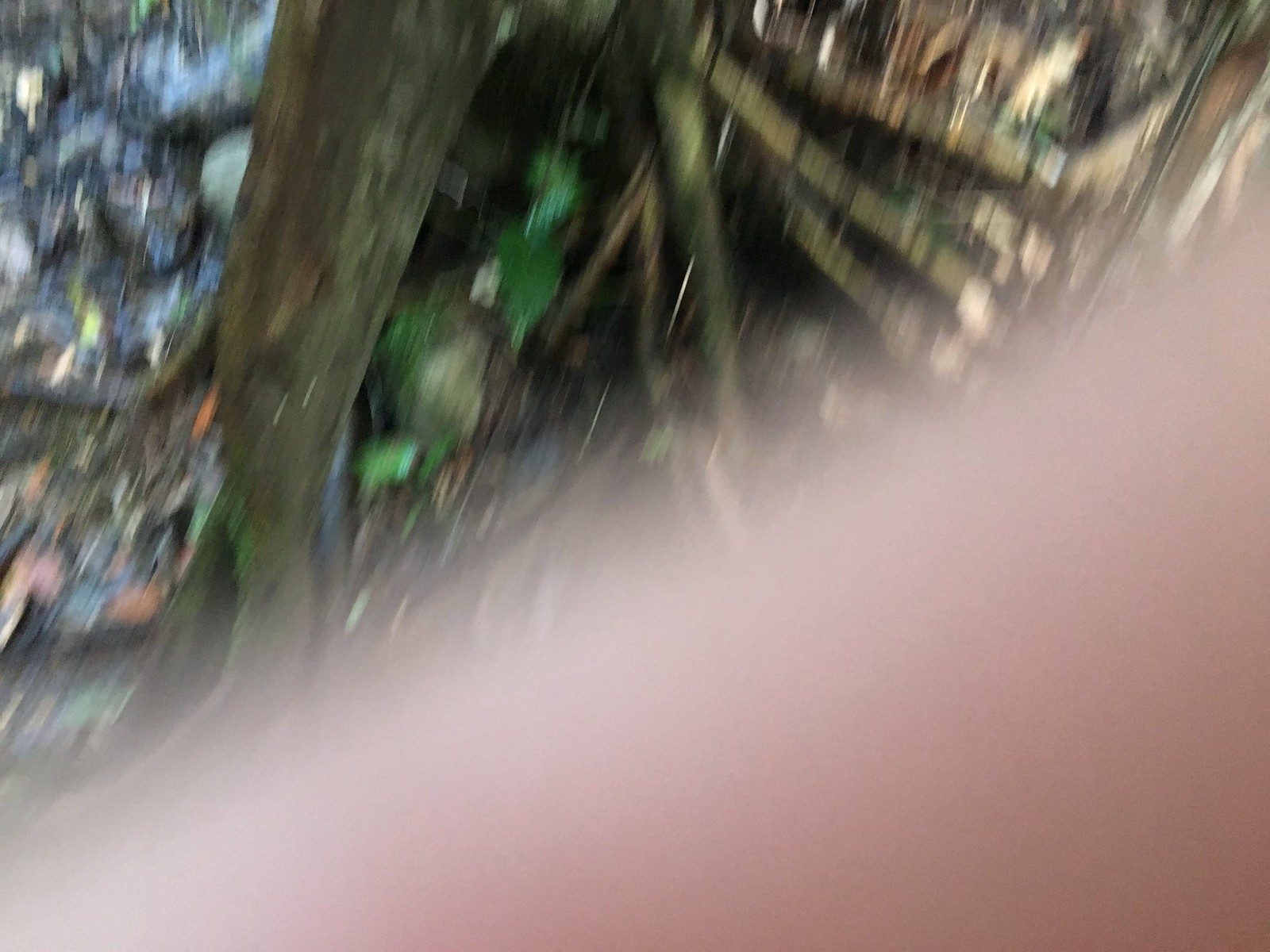In this outdoor photograph, the bottom right diagonal section is partially obscured by a light-colored finger from the person taking the picture. The remaining visible portion features a tree with extensive, sprawling roots, situated in a forested area. The forest floor is a mix of leaves and mud, indicative of a dense woodland environment, possibly along a trail. The image suffers from motion blur, resulting in a low-quality and somewhat ambiguous snapshot of a natural setting.